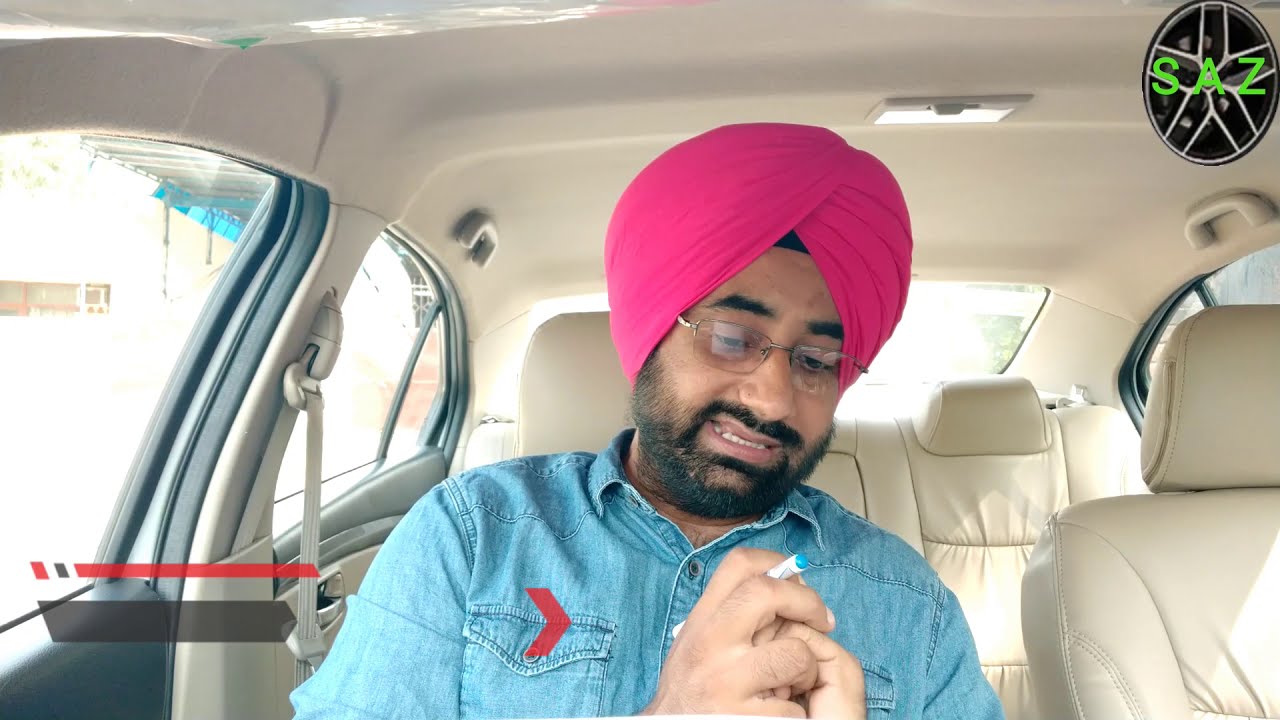In the center of this image, an Indian man is captured sitting in the driver's seat of a car on a bright day. He is adorned with a pink headscarf and glasses, and is looking down at his hand, which appears to be holding a pen. He's wearing a denim shirt with a red arrow design. The man has a beard and is not wearing a seatbelt. The interior setting of the car is visible, though the external surroundings are not, hinting it is parked. The top right corner of the image features text that reads "S.A.Z." with a red and black line beneath it. The colors predominantly visible in the image include white, pink, red, black, light green, gray, and tan.